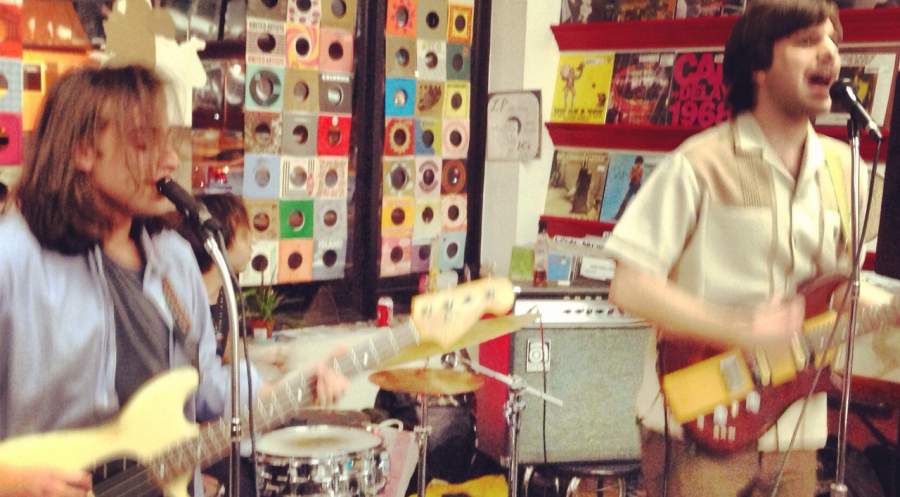In this vibrant, full-color photograph taken indoors under artificial lighting, we observe two young Caucasian males performing with guitars in what appears to be a music store or a garage setting filled with musical memorabilia. The image, although horizontally oriented and featuring no specific borders, is completely out of focus, rendering finer details indistinguishable. To the left, one male with long reddish-brown hair is wearing a blue t-shirt overlaid with a blue long-sleeved shirt. He is singing into a microphone and strumming a yellow electric guitar. On the right, the other male, sporting a beige bowling-style button-up shirt, plays a red electric guitar that has a yellow stripe down the center and sings into his microphone as well. Behind them, various musical paraphernalia, including a grey speaker and a drum set, are visible. The backdrop features a wall adorned with multiple 45s, LPs, and album shelves, adding to the busy and colorful ambiance of the scene. Despite the blurriness, the image captures a lively performance atmosphere, characterized by the musicians' joyful expressions and passionate engagement in their music.